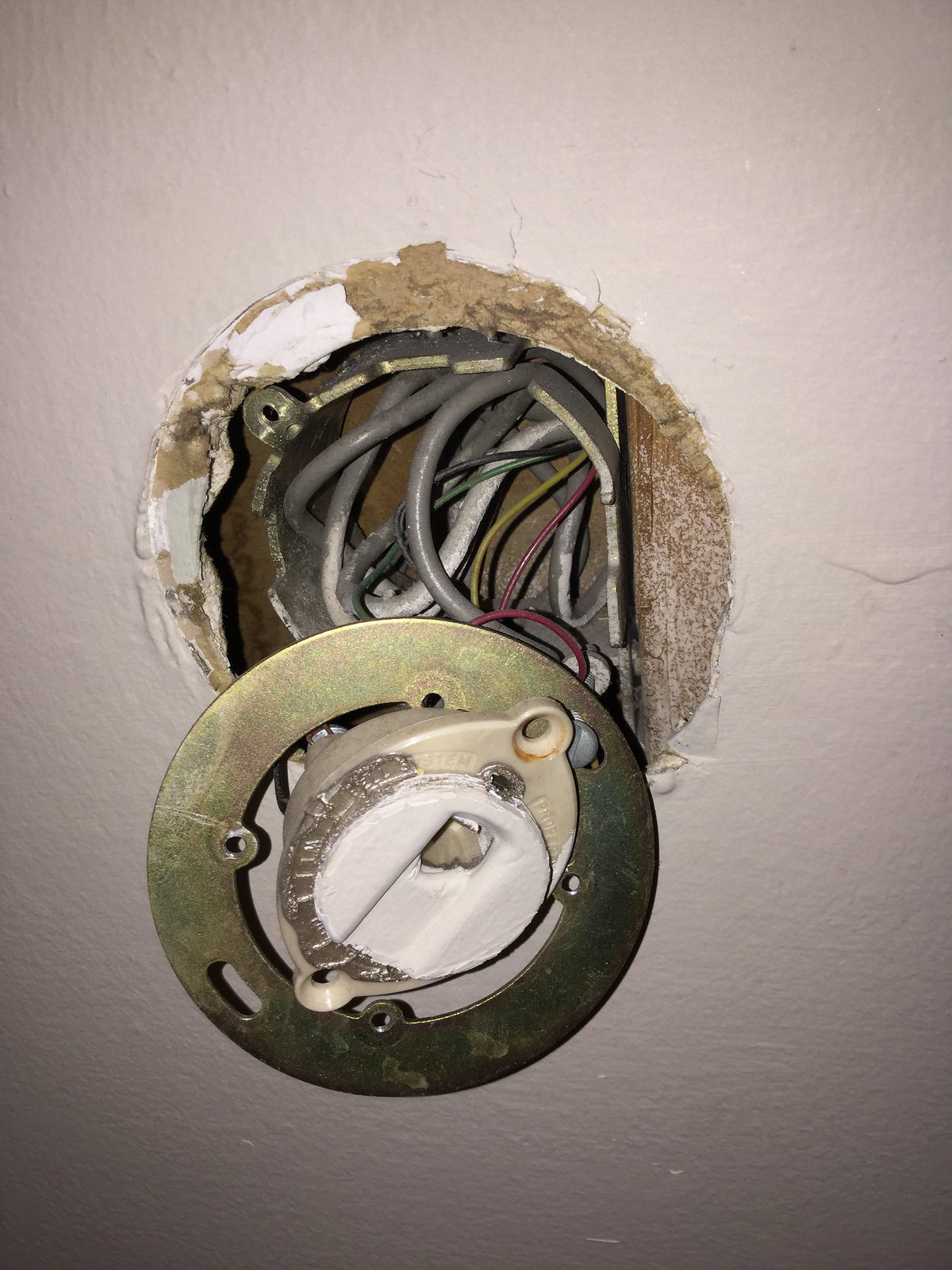A close-up image captures an aged and dilapidated doorbell affixed to a white-painted wall. The doorbell, which has a metallic, round frame, exhibits significant wear and damage, particularly in the absence of its button. Only the stump of the button remains, embedded in a once-white, now-faded circular paint mark that contrasts with the metallic frame. The frame appears dislodged, having shifted downward to expose the electrical outlet behind it. This displacement reveals an array of colorful electrical wires—gray, green, red, and yellow—amidst the brown, unpainted interior of the wall, offering a glimpse into the building’s hidden infrastructure.